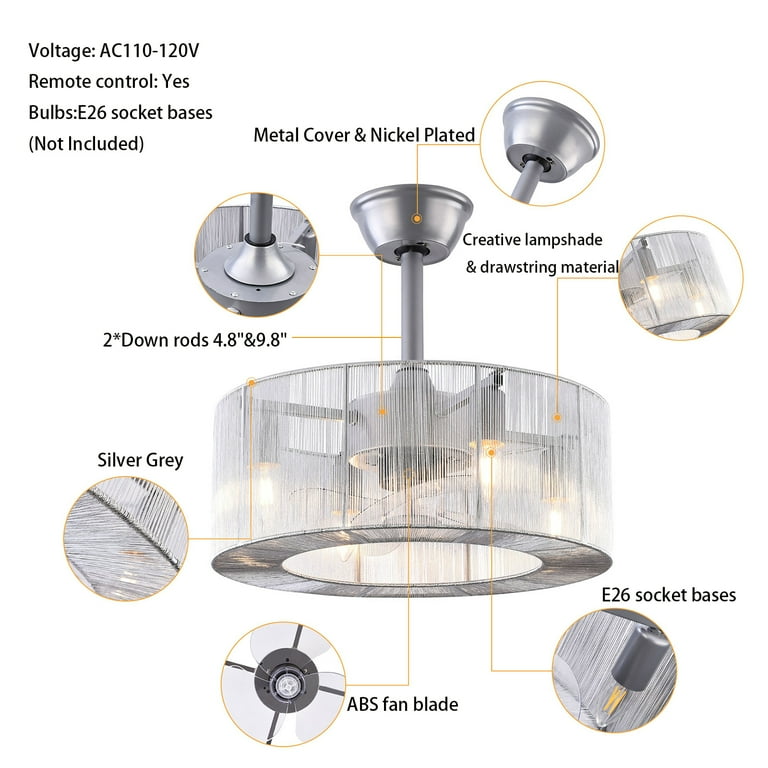The image is a detailed diagram of a silver-gray ceiling fan with a creative lampshade, meticulously labeled to show various components and specifications against a plain white background. In the upper left corner, black bold text lists key details: "Voltage AC 110-120V," “Remote Control: Yes," "Bulbs: E26 socket bases (not included)." The central part of the image is dominated by the ceiling fan, with yellow lines and circles pointing out each part. At the very top, "Metal Cover, Nickel-Plated" is labeled, indicating the section that attaches to the ceiling. Below that, a "Creative Lampshade" made of drafting materials shields the fan blades. The "E26 socket bases" are shown where the light bulbs are inserted. Arrows highlight the "ABS Fan Blade" within the lampshade and describe its structure. Another label indicates the down rods, available in two lengths: 4.8 inches and 9.8 inches. The overall diagram ensures each element, from the remote control capability to the specific materials used, is clearly identified for potential buyers.